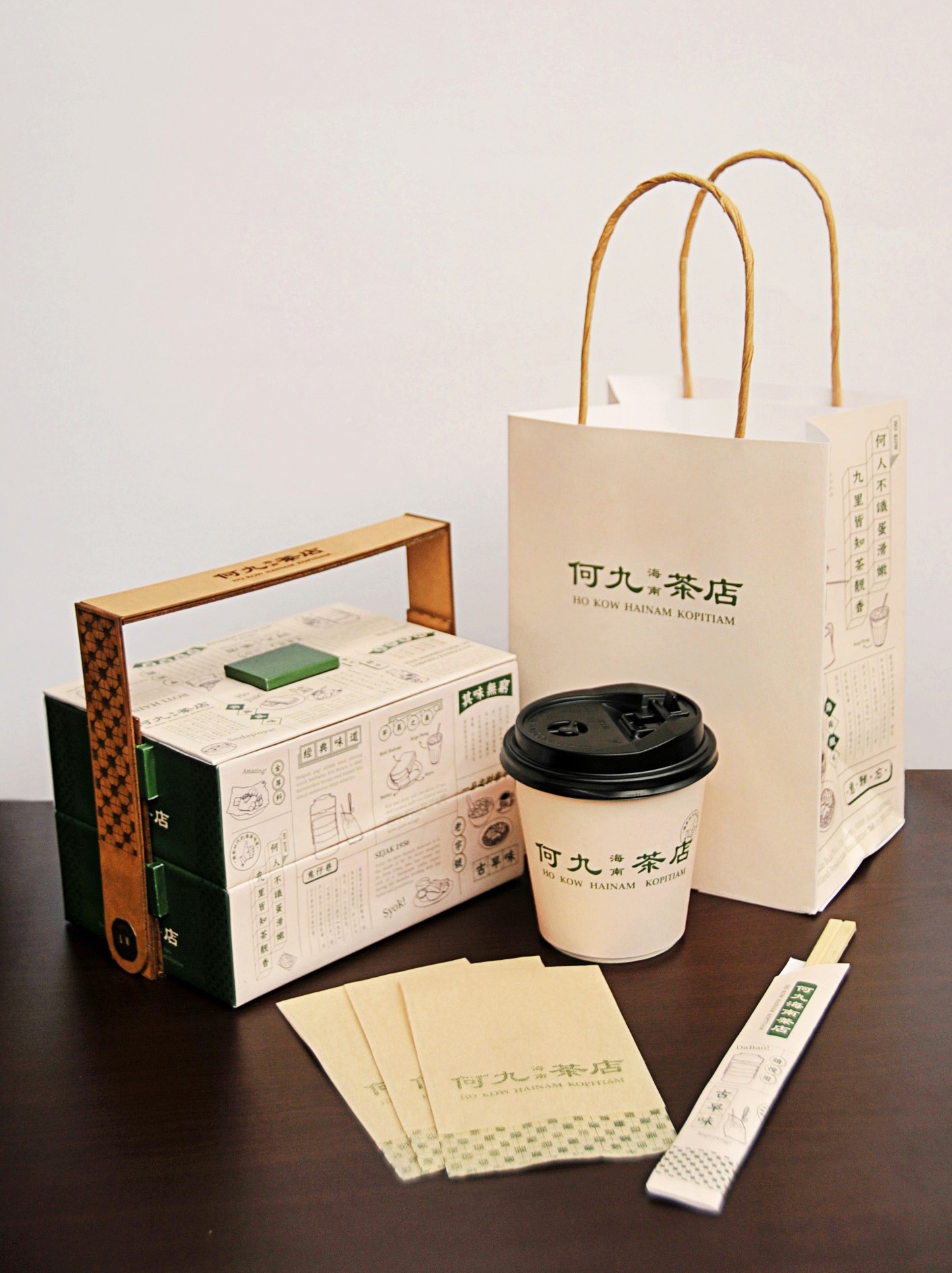The photograph features a high-gloss brown table occupying the bottom third of the image, set against a white background. On the table sits a collection of takeaway items from an Asian brand, indicated by the consistent green Chinese lettering across all items. Central to the arrangement is a white shopping bag bearing the text "Ho Kao Hainem Kopitam" in green, along with accompanying Chinese characters. In front of the bag is a white to-go coffee cup with a black plastic lid, displaying the same green text. Nearby, three light brown paper napkins are fanned out next to a pair of disposable chopsticks in a white paper sleeve. To the left of these items is a green and white to-go box with a brown square handle, likely containing food. The box seems to have instructional text, possibly detailing how to open and dispose of it, and may include nutritional information in Chinese.